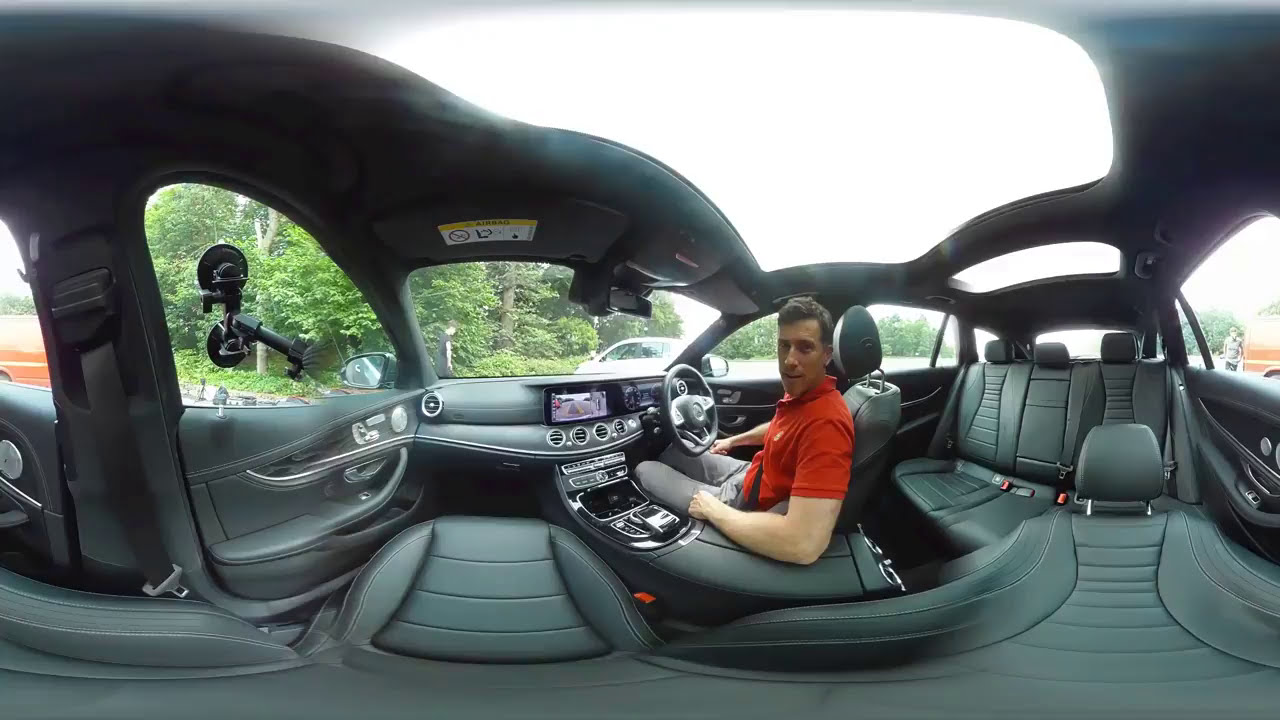A man wearing a red shirt and grey pants sits in the driver's seat of a vehicle with the steering wheel on the right side. He looks directly at the camera, while resting his elbow on the center console. The interior of the car features dark gray and black leather seats, including three seats visible behind him. Above, a large sunroof lets in bright white light, illuminating the dark interior. Outside the windows, green trees, shrubs, and a white car are visible. The image is panoramic and distorted, causing the interior to appear twisted and unnatural. Despite this, the man remains undistorted and clearly visible.